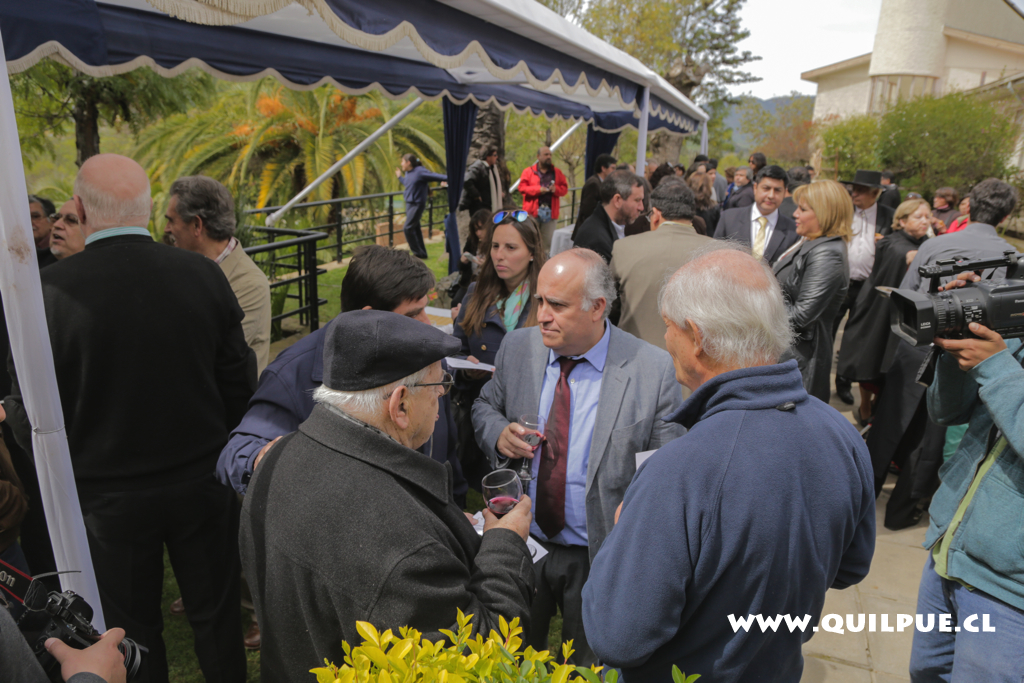The photograph captures an outdoor scene on an overcast day, featuring a crowd of people assembled around an open-air pavilion with a blue and beige canvas top. In the foreground, several men dressed in business casual attire, including suits and nice jackets, are holding drinks. One man, distinguished by his gray suit jacket, red tie, and blue collared shirt, holds a drink in his right hand. Beside him, an older gentleman wearing a flat blue hat, gray jacket, and clutching a glass of red wine in his right hand, has his back partially turned toward the camera. Another older man, with white hair balding on top but remaining around the sides and back, dons a dark blue fleece.

Among the crowd, predominantly composed of businessmen, a few women can be spotted in jackets. Notably, inside the pavilion, a young girl dressed in blue appears poised to toss a shot put, her arm raised and left leg bent in anticipation. On the right edge of the image, slightly cropped, a person operates an old-fashioned camcorder, while a white building with tall bushes can be seen in the background. Overall, this detailed scene highlights the formal gathering and various activities taking place within the outdoor setting.